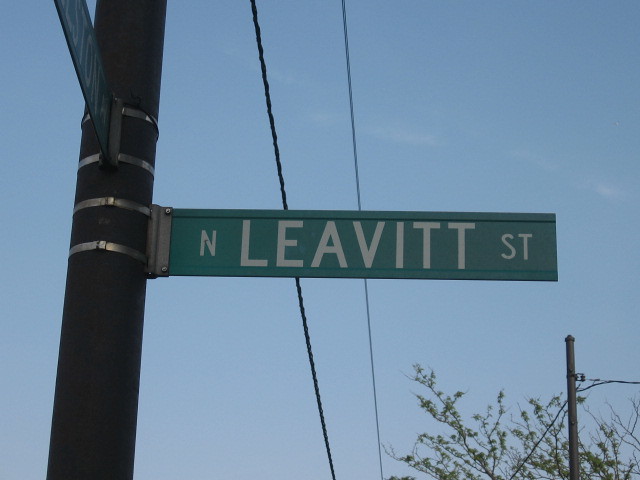The image depicts a street scene with a light blue sky on a clear, pleasant day. Centered slightly to the left within the frame, a vertical brown pole stands, angled slightly to the right. This pole features four metal clamps and supports two street signs. The prominent green street sign with off-white lettering reads "North Leavitt Street." Above it, a second sign is partially visible, but the text is unreadable as the image cuts it off. Trailing behind the street signs are two electrical wires running vertically. In the lower right corner, part of a tree is visible. The background reveals an unobstructed sky, free of clouds and people, creating a serene outdoor atmosphere.